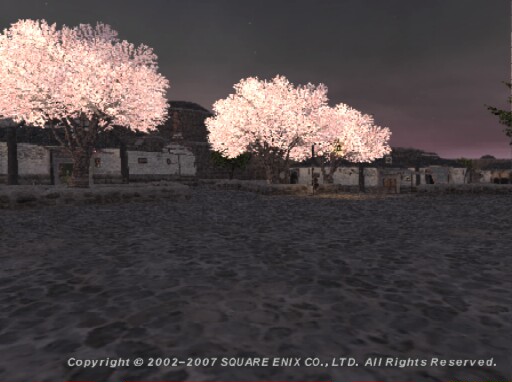The image appears to be a scene from a video game, depicting a quaint village setting. The ground is composed of stone tiles, contributing to the rustic atmosphere of the area. Stretching into the distance, there are beautiful cherry blossom trees with their pinkish hues, adding a touch of elegance to the environment. Stone structures and pathways can be observed among the trees, creating a well-defined layout of the village. In the background, houses built from white stone with dark frames around the windows and doors stand prominently. Beyond the village, a mountain looms, adding depth and a natural boundary to the scene. To the right, a verdant tree provides additional greenery. The sky above is a gradient of colors, shifting from a dark purple at the top to a lighter purple towards the bottom and right. The entire image has a subdued tone, indicative of early evening or dawn. At the bottom, there's a watermark that reads, "copyright 2002-2007 Square Enix Co. LTD all rights reserved," identifying the creators and preserving the game's intellectual property rights.